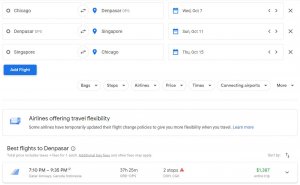The image is a promotional material for an airline detailing various flights and their schedules. It is divided into three main sections. The first section lists flights from Chicago to a destination that is not clearly visible, dated Wednesday, October 7th. The second section highlights a flight from an indeterminate location to Singapore on October 11th. The third section mentions a return flight from Singapore to Chicago on Thursday, October 15th. 

Additionally, there are seven drop-down menus related to various categories, though their specific labels are too small to discern. A notable feature of the image is a small, blocked-off window with a blue icon announcing that some airlines have temporarily updated their flight charge policies to provide greater flexibility for travelers, accompanied by a "Learn More" link.

The image also lists the best flights to a destination that appears to be "Denpor" or possibly "Densapor," with flight times ranging from 7:50 PM to 9:26 PM and a displayed price of $1,167.

Overall, the image is small and the text appears cluttered, with many details difficult to decipher.